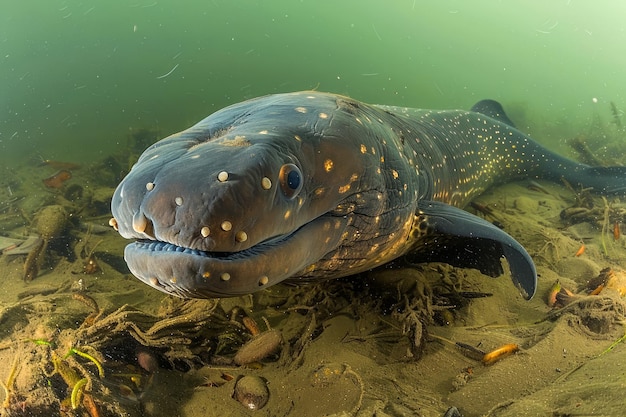The underwater image captures a murky Aussie lake with a sea creature at the center of attention. The water is a dirty green-blue, filled with sediments and laced with human debris like cell phones, plastic, and old fishing nets scattered across the sandy, brown lakebed. This large fish, resembling a miniature whale or a deep-sea creature, measures about four feet in length, comparable to the size of a small person. It has a dark navy to gray body adorned with white spots and bumps, giving it a speckled appearance. The fish’s facial structure is reminiscent of a short-nosed crocodile, with eyes positioned on the sides of its head. Despite its imposing size and distinctive features, including blue fins and lips, the fish does not appear to be dangerous, likely a scavenger inhabiting this polluted environment.